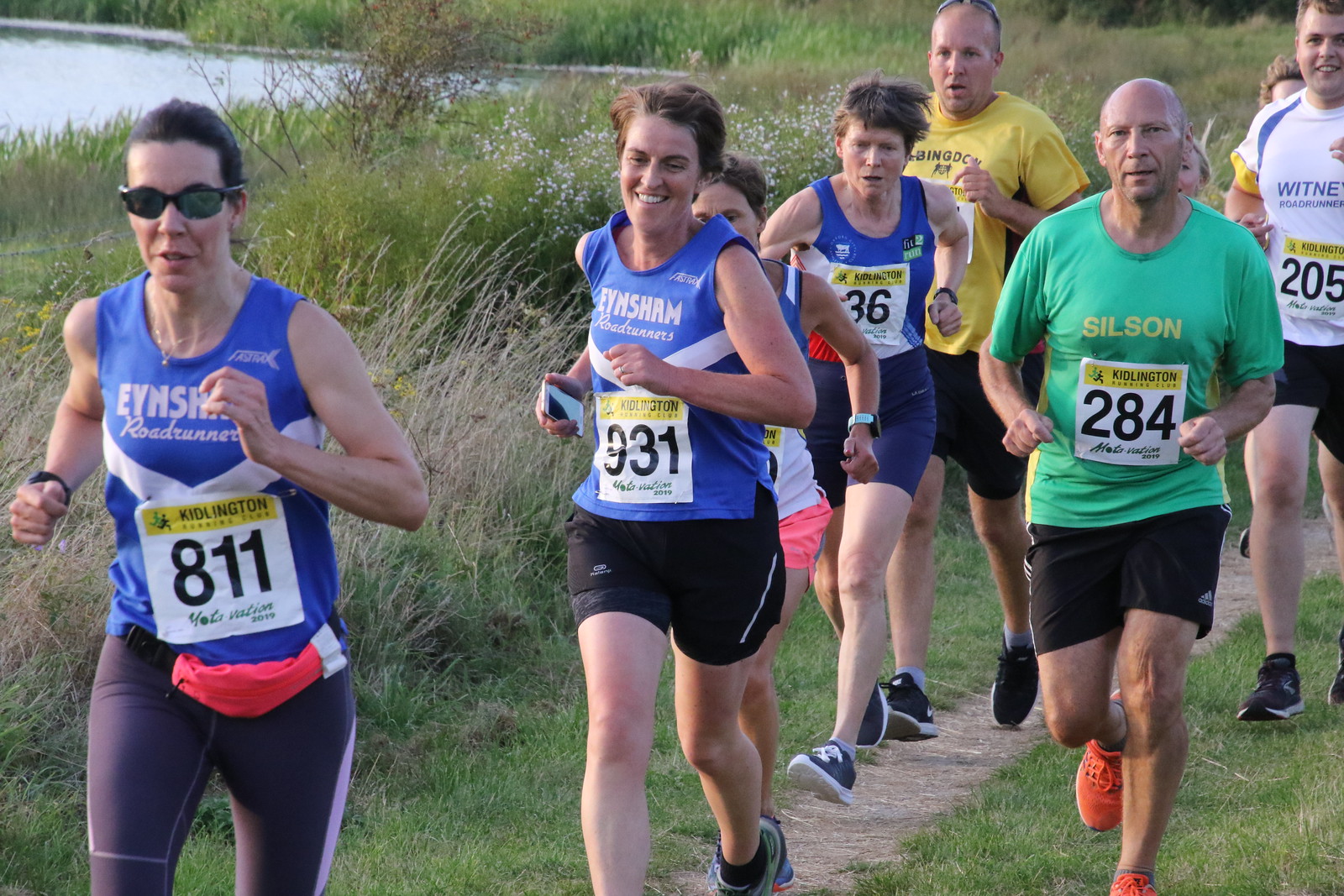In this full-color landscape photograph, a group of eight individuals is captured mid-action, participating in what appears to be a cross-country race set in a scenic, outdoor environment with abundant grass and foliage. The trail they are running on is a narrow, well-trodden path flanked by overgrown weeds and plants. A serene lake is visible in the upper left-hand corner of the image, adding to the countryside atmosphere.

Leading the pack is a woman with glasses wearing a blue top and blue pants, bearing the race bib number 811. Close behind her is another woman with a blue shirt and black shorts, marked with the bib number 931. Flanking her is a woman in a blue shirt paired with pink shorts. Following them is a bald man in a green shirt that reads "SILSON" and orange shoes, sporting the bib number 284.

Further back, a woman dressed in a blue short-sleeve shirt and blue leggings can be seen, alongside a man in a yellow shirt and black shorts. Another younger girl is partially obscured, and at the very rear, a young man with a white shirt adorned in blue trim and black shorts, wearing the bib number 205, is visible. The participants all display race number tags, hinting at an organized event, possibly taking place in late spring or early fall, as they run in what appears to be cool and comfortable weather.